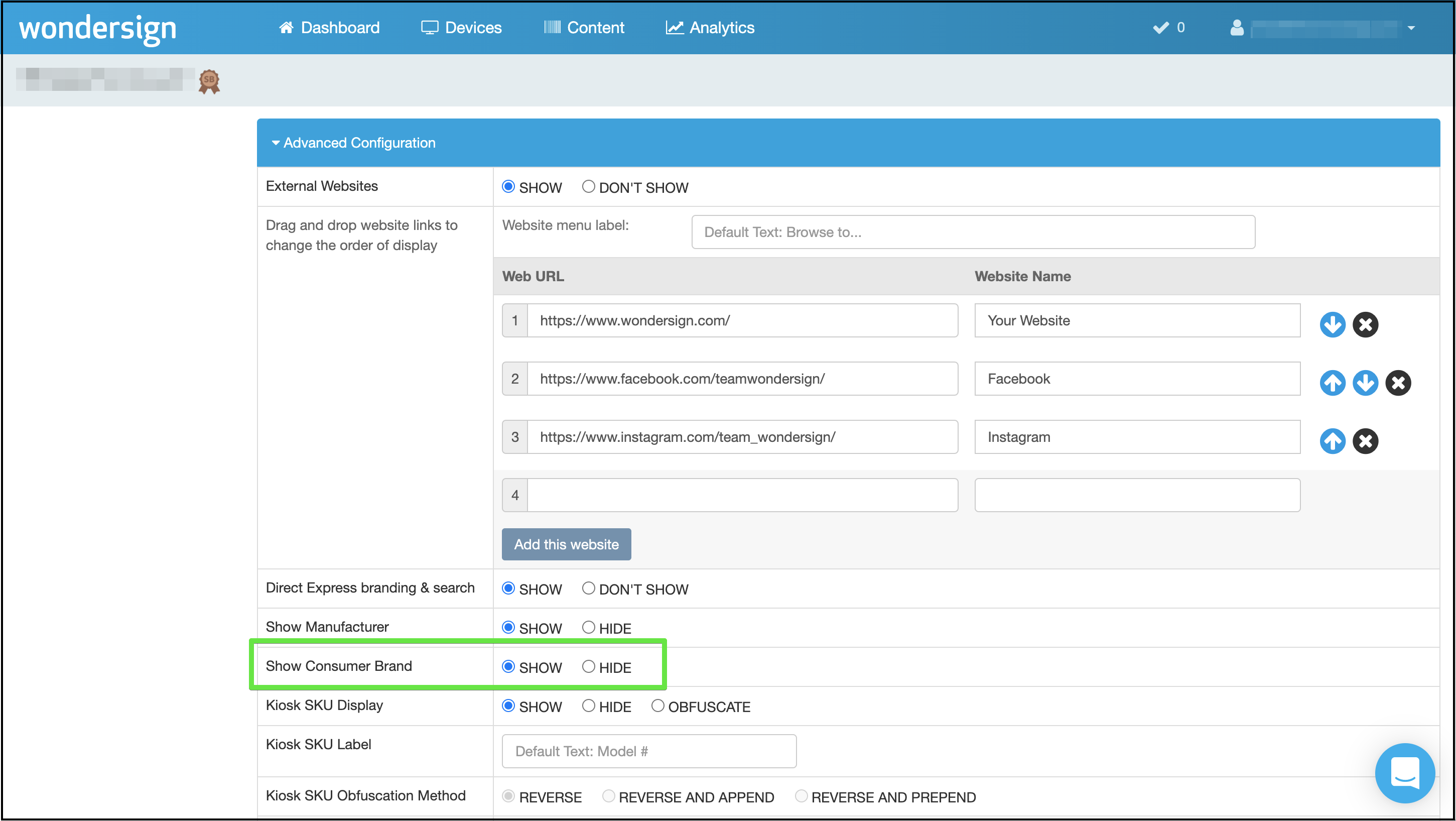The image displays a webpage with a detailed dashboard interface. In the top-left corner, there is a "Wonder Sign" label. The dashboard contains navigational sections such as Devices, Contents, Analytics, Advanced Configuration, and External Websites. A specific area on the page is dedicated to organizing website links, allowing users to drag and drop to change their display order.

Beneath the heading "Website Menu Label," the page lists several URLs: the first being "https://www.wondersign.com," the second "www.facebook.com," and the third "www.instagram.com." The term "Shoe Consumer Brand" is highlighted in green, while other visible texts mention "Direct Express Branding," "Search," "Shoe Manufacturer," as well as "Kiosk SKU Display" and "Kiosk SKU Label." This meticulous structure aids users in managing and configuring their web resources efficiently.